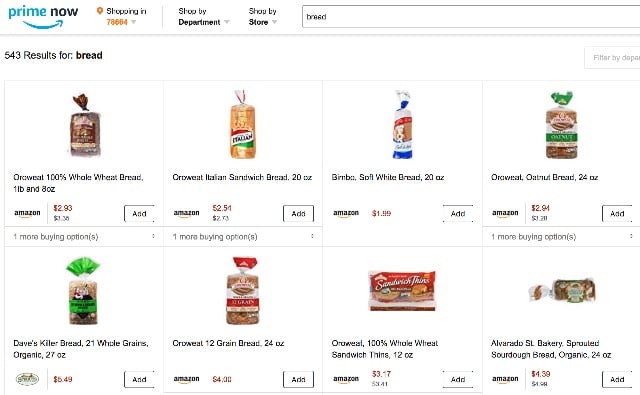This image depicts a screenshot of the Amazon Prime Now shopping interface, with a predominantly white background. In the top left corner, the text "Prime Now" is displayed, where "Prime" is in blue and "Now" is in black, accompanied by a right-pointing arrow. Below that, the location setting shows "Shopping in 78664" with a drop-down menu. The options "Shop by Department" and "Shop by Store" are visible.

At the center of the interface is the search bar with the word "Bread" typed into it. The search results below the search bar showcase a variety of bread options, each accompanied by its respective price and additional details:

1. **Oatmeal 100% Whole Wheat Bread** - 1 lb and 8 oz, priced at $2.93 (Retails for $3.30).
2. **Crow Wheat Italian Sandwich Bread** - 20 oz, available with additional details suggesting "Amazon 251" with an "Add" button next to it.
3. **Bare Boat Soft White Bread** - 20 oz, priced at $1.99.
4. **Oatmeal Oat Nut Bread** - 24 oz, priced at $2.91.
5. **Dave's Killer Bread 21 Whole Grains and Seeds, Organic** - 27 oz, priced at $6.49.
6. **Crow Wheat 12 Grain Bread** - 24 oz, priced at $4.
7. **Oatmeal 100% Whole Wheat Sandwich Bread** - 12 oz, priced at $3.17.
8. **Alvarado St. Bakery Sprouted Sourdough Bread, Organic** - 24 oz, priced at $4.39.

Each bread option has its own distinct details and price, providing the user with various choices for their bread purchase on the Amazon Prime Now platform.